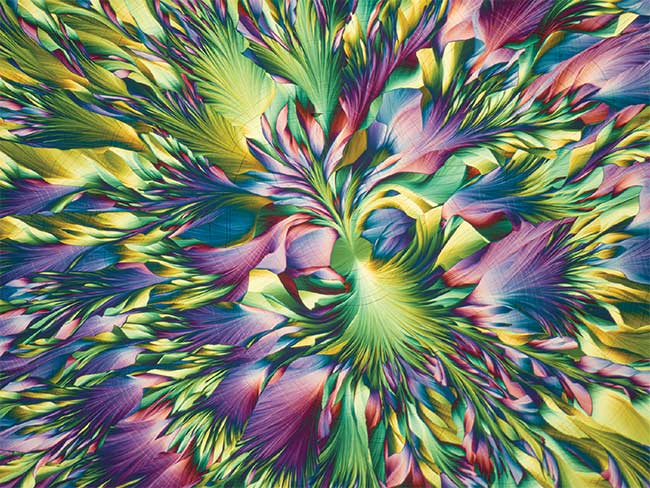The image is an animated abstract drawing depicting a vibrant, feather-like arrangement with a rich palette of Mardi Gras-inspired colors—green, purple, blue, yellow, and pink, with occasional hints of white and lavender. The composition features numerous feather-like objects that are densely clustered around the edges and more sparsely positioned towards the center. The central element of the image is a prominent large green feather or flower, surrounded by other smaller feather-like forms. While the overall distribution does not follow a precise pattern, it has a deliberate and artistic layout that creates a dynamic visual effect. The rendering is done in a manner that could suggest the use of paint, markers, or colored pencils, and gives an impression of either floral motifs or feathers as seen from a distance. The abstract nature of the piece, combined with its vivid and varied colors, enhances its intricate and harmonious design.